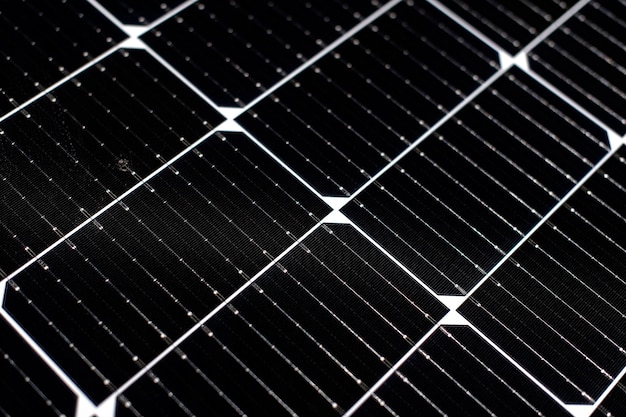The image features a highly detailed, close-up view of a metal grate. The photograph is presented in a vertical rectangular format, focused solely on the intricate design of the grate without any background context. The main structure comprises thinner silver wires that stretch diagonally from the upper left to the lower right. Intersecting these are thicker, stronger silver cables forming a pattern that extends from the bottom left to the top right, creating a series of elongated, rectangular shapes with a bright silver hue, contrasting against the softer, thinner wires.

Additionally, there are faint diagonal lines traveling from the top left to the bottom right, contributing to a grid-like appearance. This intricate web of lines and rectangles sits atop a darker, gunmetal or very dark silver background, which is less reflective than the silver wires. The overall design resembles a network of shimmering, lucid lines akin to spider silk or wires adorned with water droplets, giving the structure a glossy, almost new appearance.